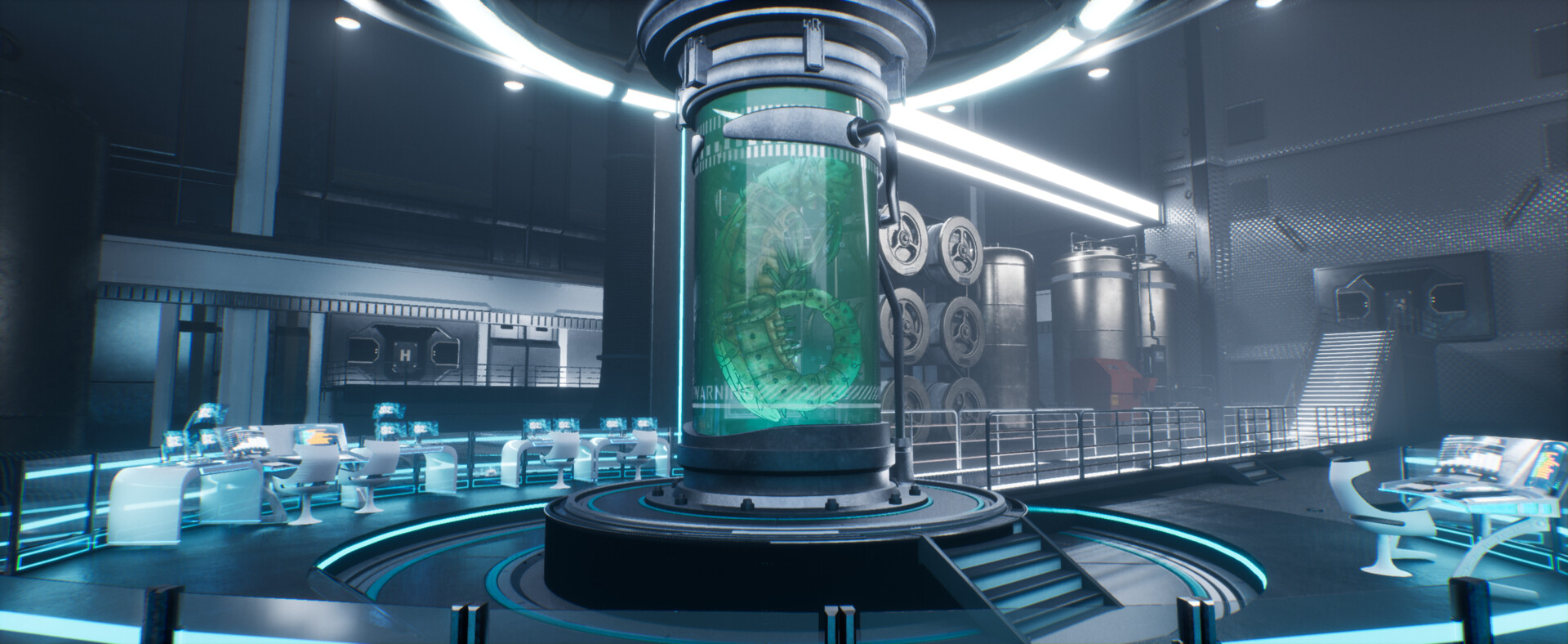The image depicts a detailed, futuristic scientific laboratory, meticulously crafted to resemble a high-tech sci-fi facility. Dominating the foreground is a large, green fluid-filled tank with an indistinct creature, exuding an aura of extraterrestrial mystery. Surrounding the tank are advanced computer workstations and space-age chairs, all bathed in the cool glow of LEDs and blue light emitted from the sophisticated equipment. The room is adorned with various scientific apparatus, including bottles, wheels on the walls, and tanks that likely store fluids or gases. The lab's aesthetic is defined by its sleek black, blue, green, and white color palette, paired with the reflective sheen of silver and dark silver surfaces. Fluorescent lighting adds to the clinical yet otherworldly atmosphere. There are small stair steps leading to the tank, as well as additional stairs heading to an adjoining room, perhaps another part of this expansive futuristic facility. Though devoid of people, the image hints at a space designed for meticulous scientific observation and experimentation, reminiscent of an elaborate digital rendering rather than a photograph, possibly created using advanced software like Adobe Photoshop.